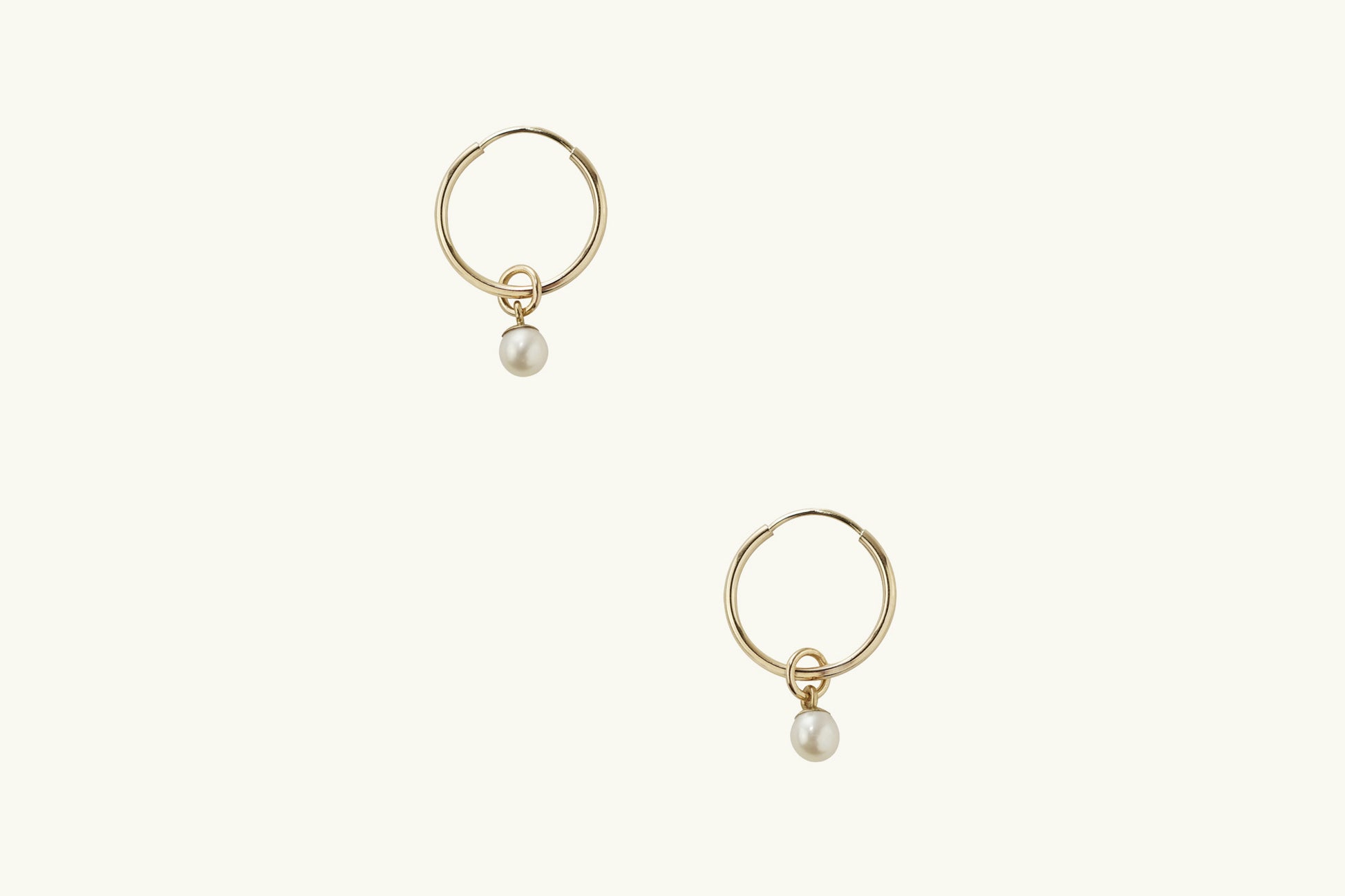The image displays a pair of exquisite golden hoop earrings set against a creamy, off-white background. Each earring consists of a larger gold hoop featuring a hinged mechanism for securing it. From this larger hoop hangs a smaller gold hoop, and connected to the smaller hoop is a delicate pearl with its own tiny hoop. The earrings, identical in style, are beautifully understated and delicate, with one positioned in the upper left and the other in the bottom right of the image. The simplicity of the background draws all attention to the elegant craftsmanship and detail of the earrings, suggesting they may be showcased in an advertisement for a jewelry store.